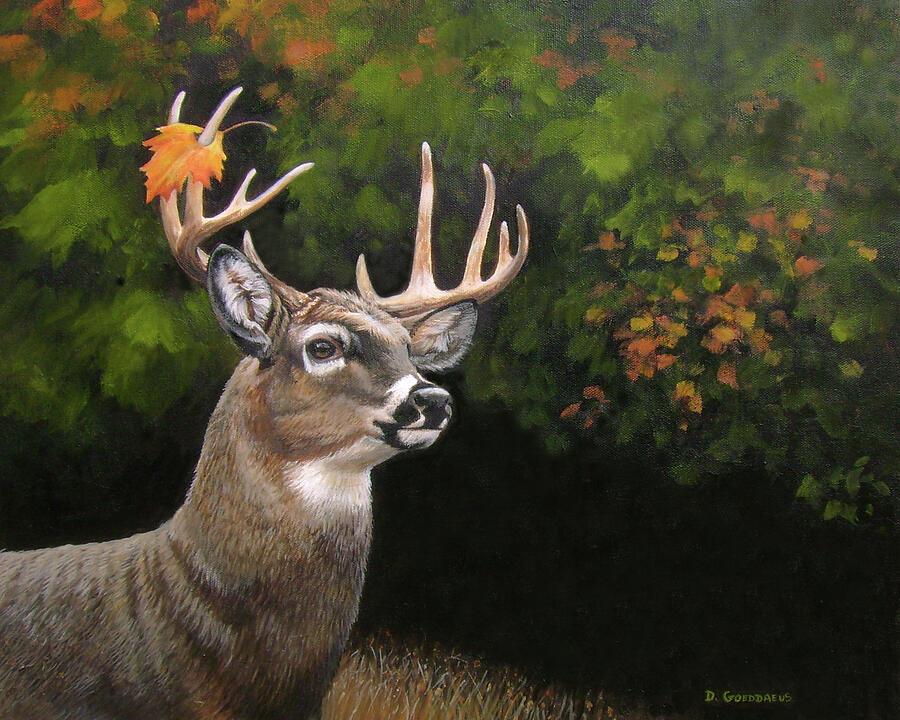This is a detailed painting by D. Godarius depicting a majestic deer in a vibrant autumn setting. The deer, with its brown and white fur, stands prominently in the foreground, gazing intently to the right. Its large, intricate antlers catch the attention, particularly one antler that's pierced through by a yellow-orange fall leaf. You can see only one of the deer's eyes, emphasizing its focused yet serene expression. The background features a forest with a mix of green, yellow, and orange leaves, indicating the early stages of autumn. Tall grasses surround the deer, creating a natural frame. The painting employs oil technique, showcasing a stunning mix of blurred and detailed elements, bringing the entire nature scene to life.